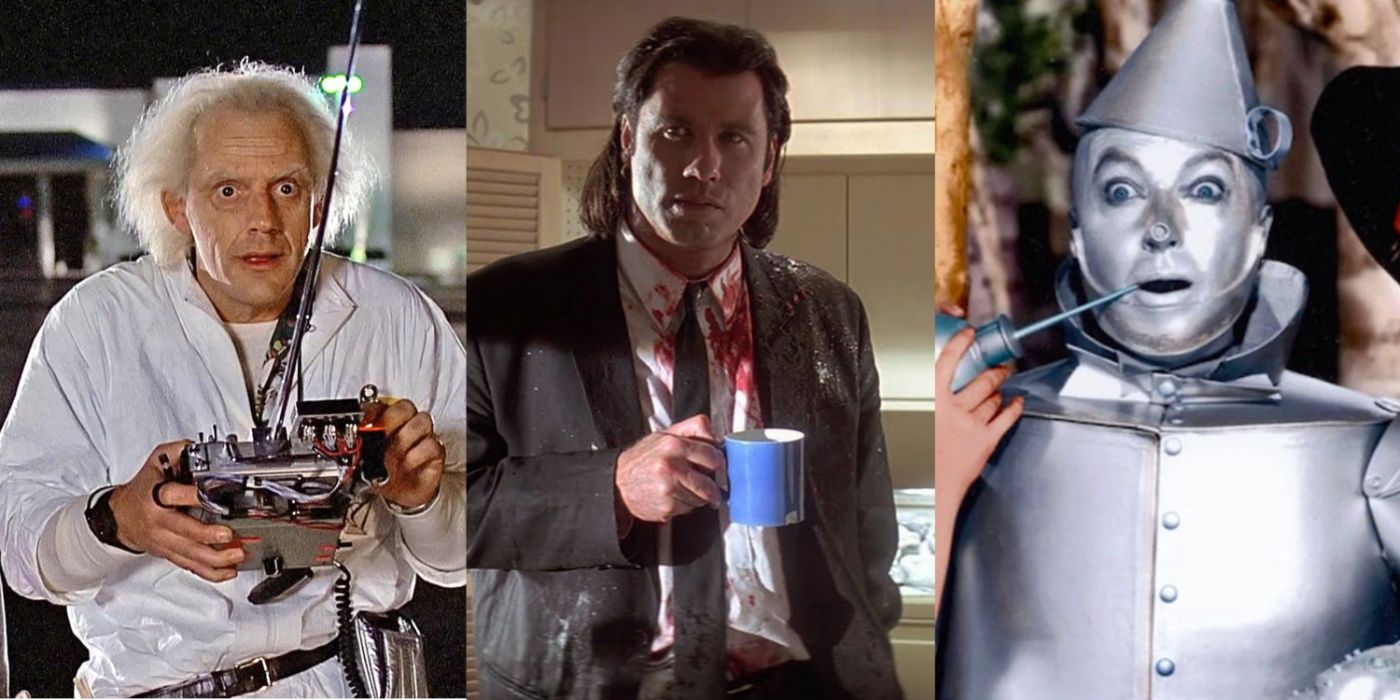This collage features three iconic characters from classic films aligned side by side. On the left is Doc Brown from the Back to the Future series, holding a remote control with intricate wires and an antenna, wearing a white, long-sleeved top and sporting wild, long gray hair. The center image portrays John Travolta in Pulp Fiction, donning a black suit with a white shirt and black tie, both stained with blood, as he holds a blue coffee mug and gazes to the left. On the right stands the Tin Man from The Wizard of Oz, clad in his metallic suit and silver-painted face, with Dorothy using an oil can to lubricate his mouth so he can move again. The Scarecrow's hat is also visible next to the Tin Man.